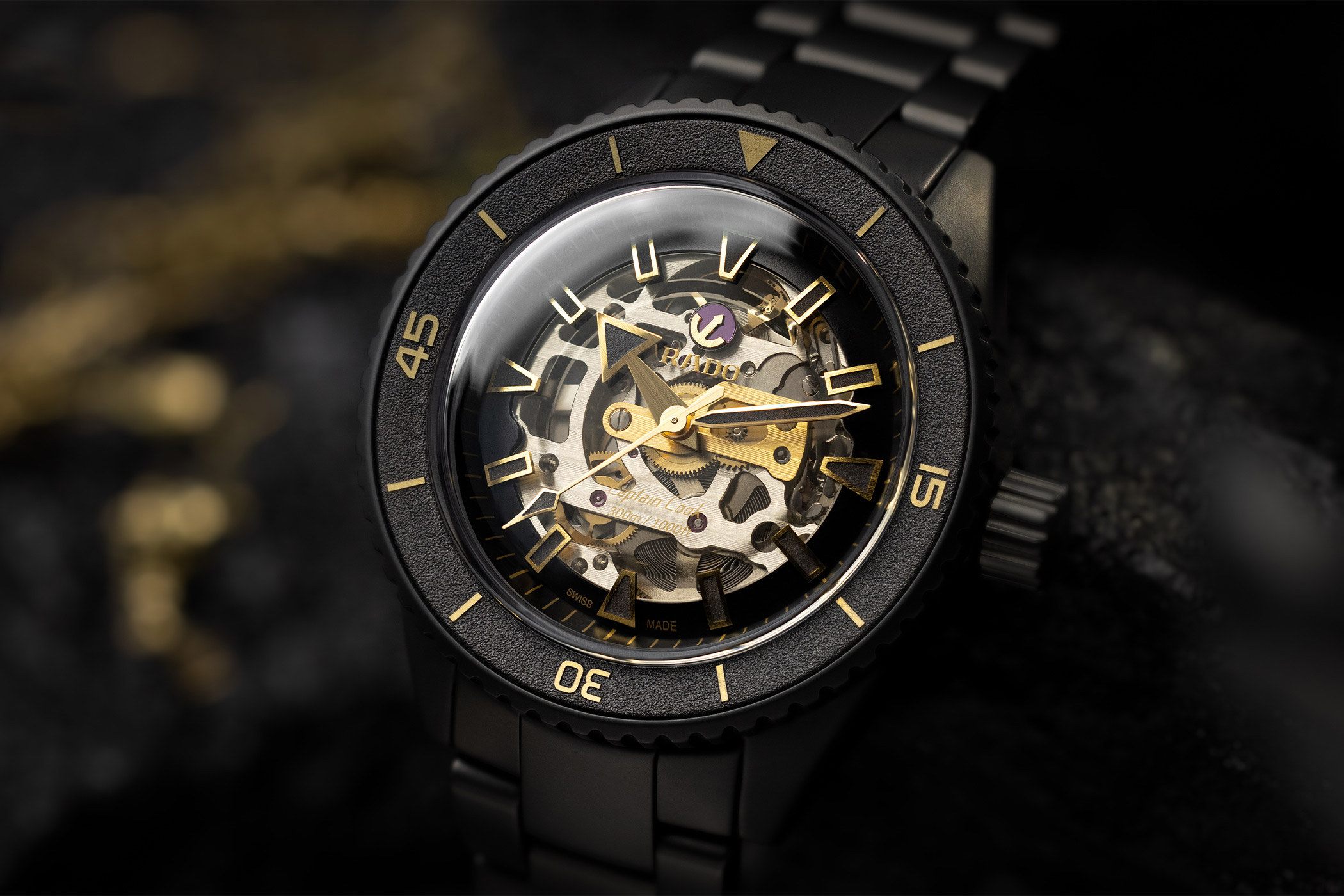This image features a luxury watch, prominently showcasing its intricate inner workings through a clear glass face. The watch is primarily black with elegant gold accents, including gold numbers and hour markers, and a black band. The minute and hour hands are gold with black detailing, while the second hand is entirely gold. The minute markers, labeled 15, 30, and 45, are clearly visible around the perimeter. At the 12 o'clock position, there is a small purple square housing a gold anchor, which is part of the Rado brand logo. The brand "Rado" is printed in gold at the center of the watch face, just above the inscription "Captain Cook 300M / 1000 feet." A black knob is located on the side of the watch. The background of the image is primarily black and blurred, focusing attention on the detailed and exquisite craftsmanship of the watch.